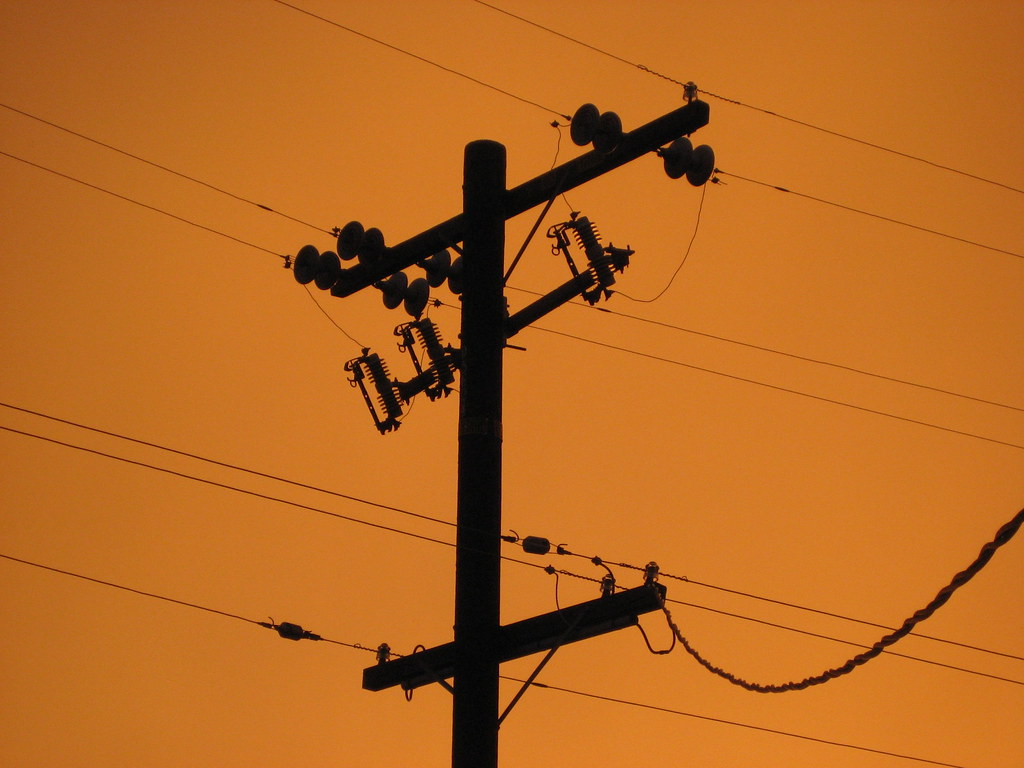The photograph depicts a stark, black silhouette of a utility pole against a vibrant reddish-orange sky, likely captured during a dramatic sunset or under unique lighting conditions. The utility pole, originating from the bottom center and extending almost to the top of the rectangular, 6-inch wide by 4 to 5-inch high image, features three horizontal crossbars. The lowest crossbar supports a thick wire that curves downward and to the right, while the upper two crossbars bristle with numerous wires. Most of the wires stretch from the upper left to the lower right, with the seven most prominent wires arranged in pairs, except for the last solo wire at the bottom. Each wire connects to the pole via cylindrical, disc-shaped insulators, although the insulators themselves are mostly obscured by shadows. Additionally, several rectangular boxes are affixed to the pole, one on the right and two on the left. Shadows cast by the pole and its attachments render all elements uniformly black, accentuating the vivid, monochromatic contrast between the silhouetted pole and the fiery background.